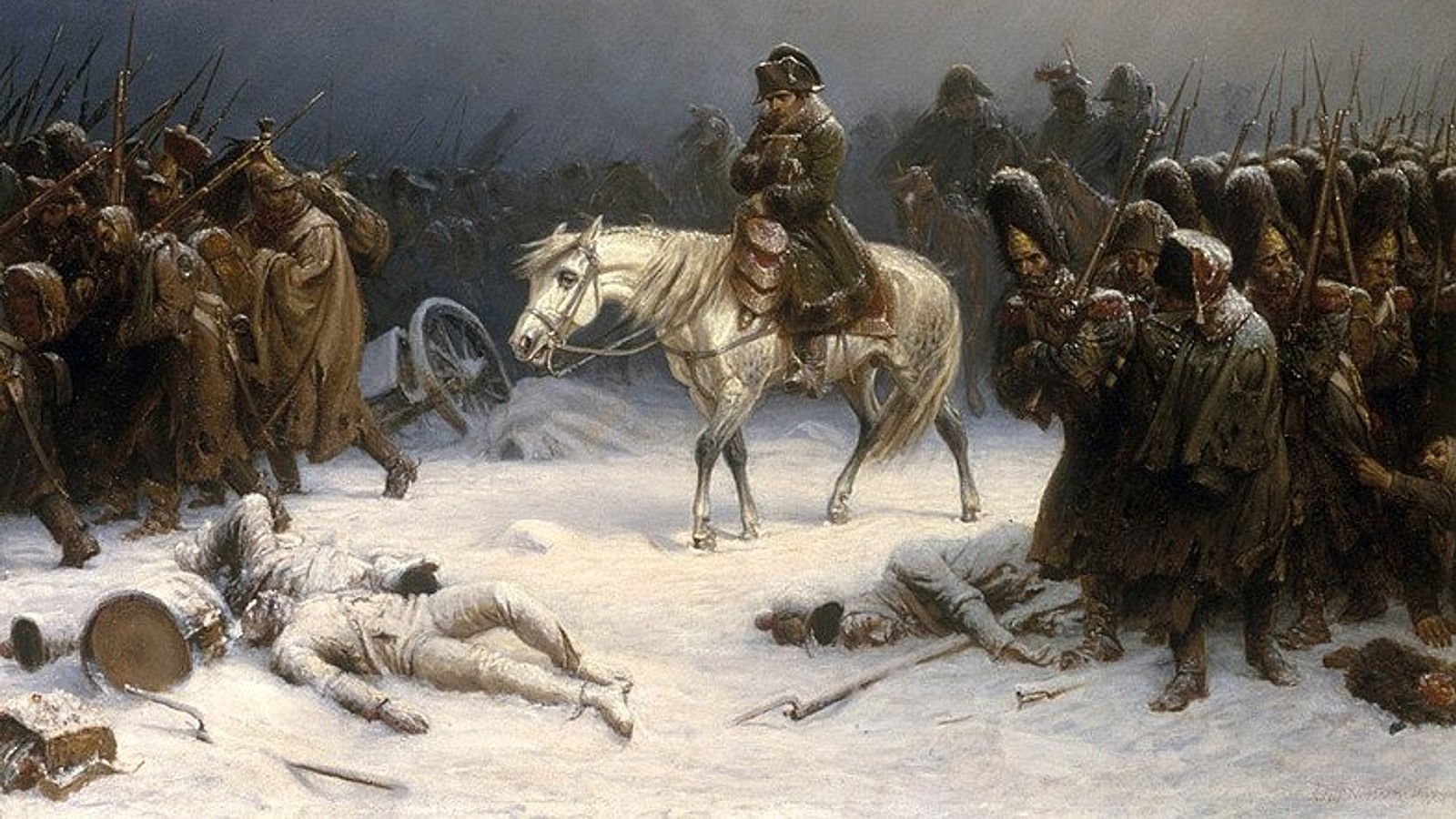The image depicts an old painting showcasing a wartime scene set in a snowy landscape. At the center is a man, likely a general, riding a tired white horse, donning a uniform complete with a coat and hat. Surrounding him are numerous soldiers carrying muskets, trudging through the snow. The ground is littered with fallen soldiers, their bodies partially covered by the snow, alongside scattered rifles. In the background, there is a tipped-over carriage wheel, adding to the chaotic aftermath of the battle. The sky above is hazy and gray, casting a somber tone over the entire scene.